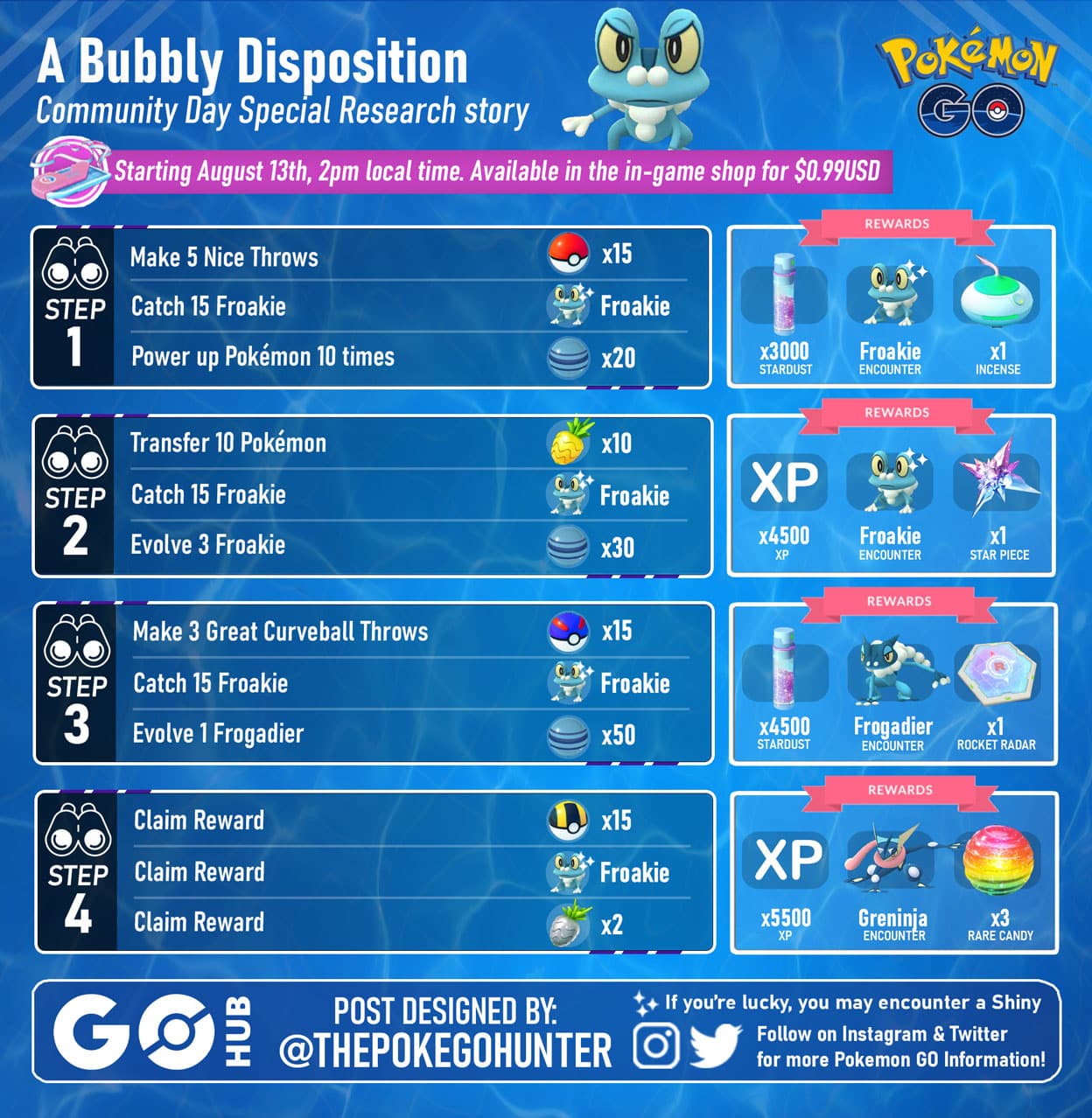This image features a promotional advertisement for a Pokémon GO Community Day Special Research Story event. The background is a gradient of light and dark blue hues, setting a vibrant and eye-catching scene. At the top, in white bubble-style lettering, it states, "I have a bubbly disposition, community day special research story." Below this text, there is an illustration of a cheerful, animated frog Pokémon.

The iconic Pokémon GO logo is prominently displayed, with the letters "G" and "O," and the word "GO" underlined. A purple banner indicates the event's details: "Starting August 13th, 2 PM local time, available in the game shop." It appears to be a special in-game purchase or offer exclusive to Community Day.

The layout includes a structured four-step research task list, each step featuring three specific tasks. These tasks seem to offer various in-game rewards upon completion. To the right, the potential rewards are clearly detailed, showcasing items such as Stardust, Pokémon encounters, Incense, XP, and more, enhancing the appeal of participating in the event.

At the bottom of the advertisement, there's a credit line stating, "Designed by Ad, the Poké GO Hunter" and a call-to-action to follow the event on social media platforms for more updates. The footer also mentions the potential to encounter a Shiny Pokémon, adding an extra layer of excitement for fans. Social media icons for Instagram and Twitter are provided for easy access to follow Pokémon GO International updates.

Overall, the image acts a comprehensive and engaging invitation for Pokémon GO players to join the upcoming Community Day event.